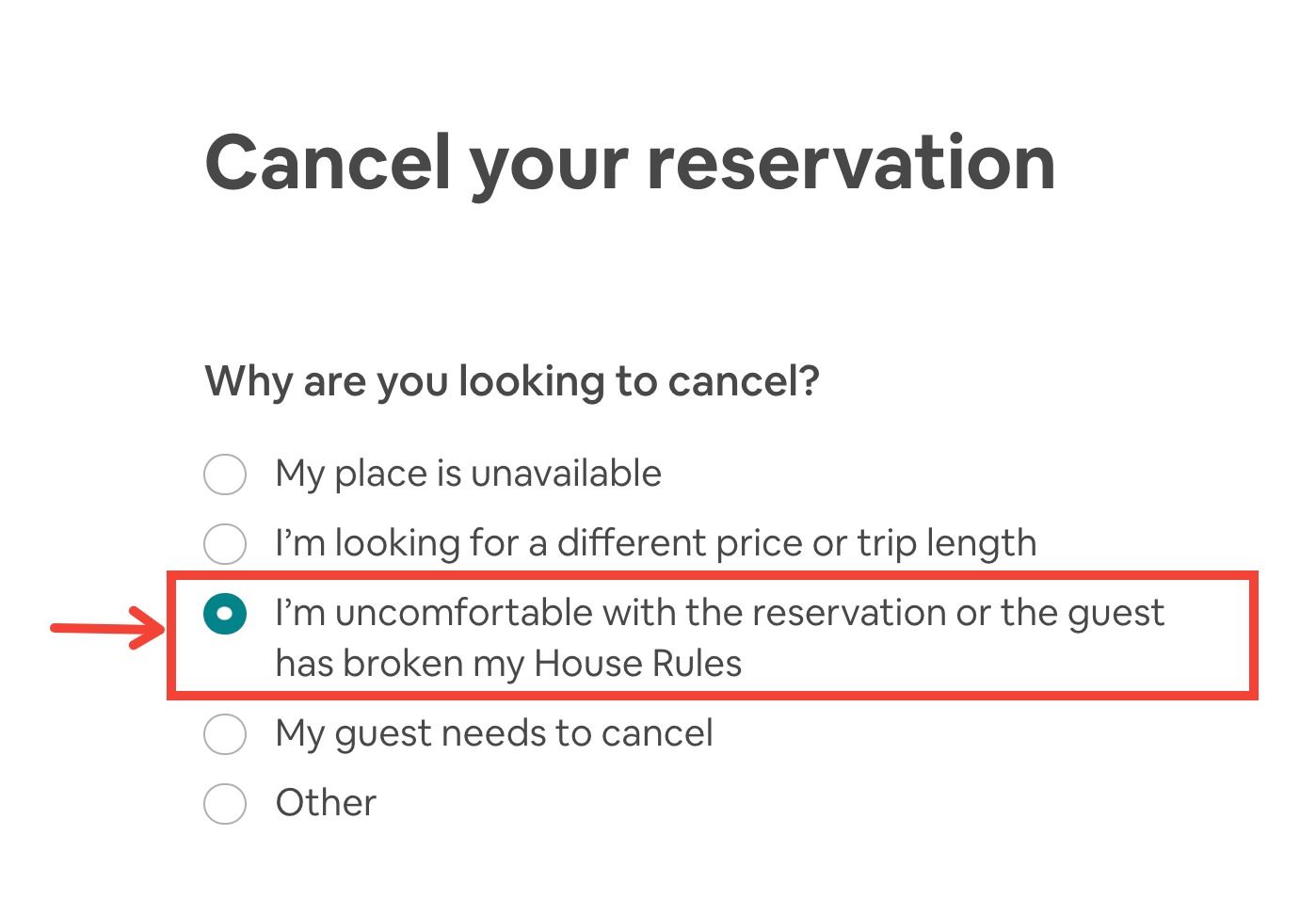The image displays a screenshot of a reservation cancellation interface, presented on a solid white background. At the top center, bold dark gray text reads "Cancel Your Reservation." Following a noticeable space, there is a line of smaller text that asks, "Why are you looking to cancel?" Beneath this question are five light gray-outlined circular options for selecting the reason for cancellation. 

The first option states, "My place is unavailable." 
The second option reads, "I'm looking for a different price or trip length."
The third option, highlighted with a teal fill and red outline, shows an arrow pointing to it and indicates, "I'm uncomfortable with the reservation or the guest has broken my house rules."
The fourth option says, "My guest needs to cancel."
The fifth and final option lists, "Other."